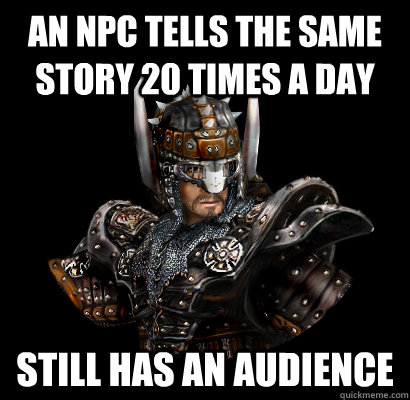In the photograph, a heavily muscular, bald white man with a grayish beard and mustache is perched on a bed in an almost gorilla-like pose. His flexed triceps and tattooed right shoulder are prominently displayed. The man, seen from his right side, wears a black and grey belt with a strap across his right thigh, possibly part of a jockstrap or lingerie. A black cylinder-like object with a white band wraps beneath his legs, adding to the provocative nature of the scene. The bedspread is a striking camouflage pattern in shades of gray, black, white, and red, complemented by two black pillows with white lines. Behind him, the wall is a muted grey. The image is completed by the text "HAI" centered at the bottom, greeting the viewer with the bold, capitalized letters. The man’s piercing gaze adds to the intense and sexually suggestive composition of the photograph.